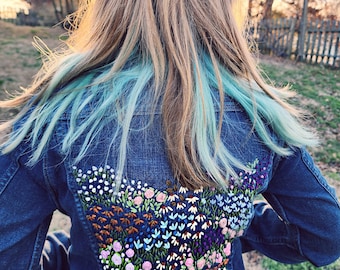In a vibrant backyard setting, a young woman stands with her back to the camera, highlighting her striking appearance and attire. Her long, shoulder-length blonde hair cascades down, with the top layer a soft blonde that transitions into shades of brown, and the bottom portion, about six to eight inches at the nape of her neck, dyed a light blue or teal green. She wears a long-sleeve blue denim jacket adorned with an intricate and colorful embroidery of flowers, which serves as the focal point of the photo. The floral design on the jacket features a variety of colors: white flowers in the upper left, sunflowers above with pink flowers to the left, orange flowers clustering on the left, pink ones beneath them, light blue in the center, more pink flowers in the lower right, small purple flowers just above these, and another mix of orange and light blue flowers higher up. The detailed embroidery captures a delightful palette, including pink, blue, orange, and yellow, making the jacket an eye-catching piece. She stands seemingly at ease with her hands in her pockets within a yard characterized by its mostly brownish-green grass, a wooden fence visible in the upper right background, and a hint of trees with sunlight filtering through in the distance, enhancing the serene atmosphere.